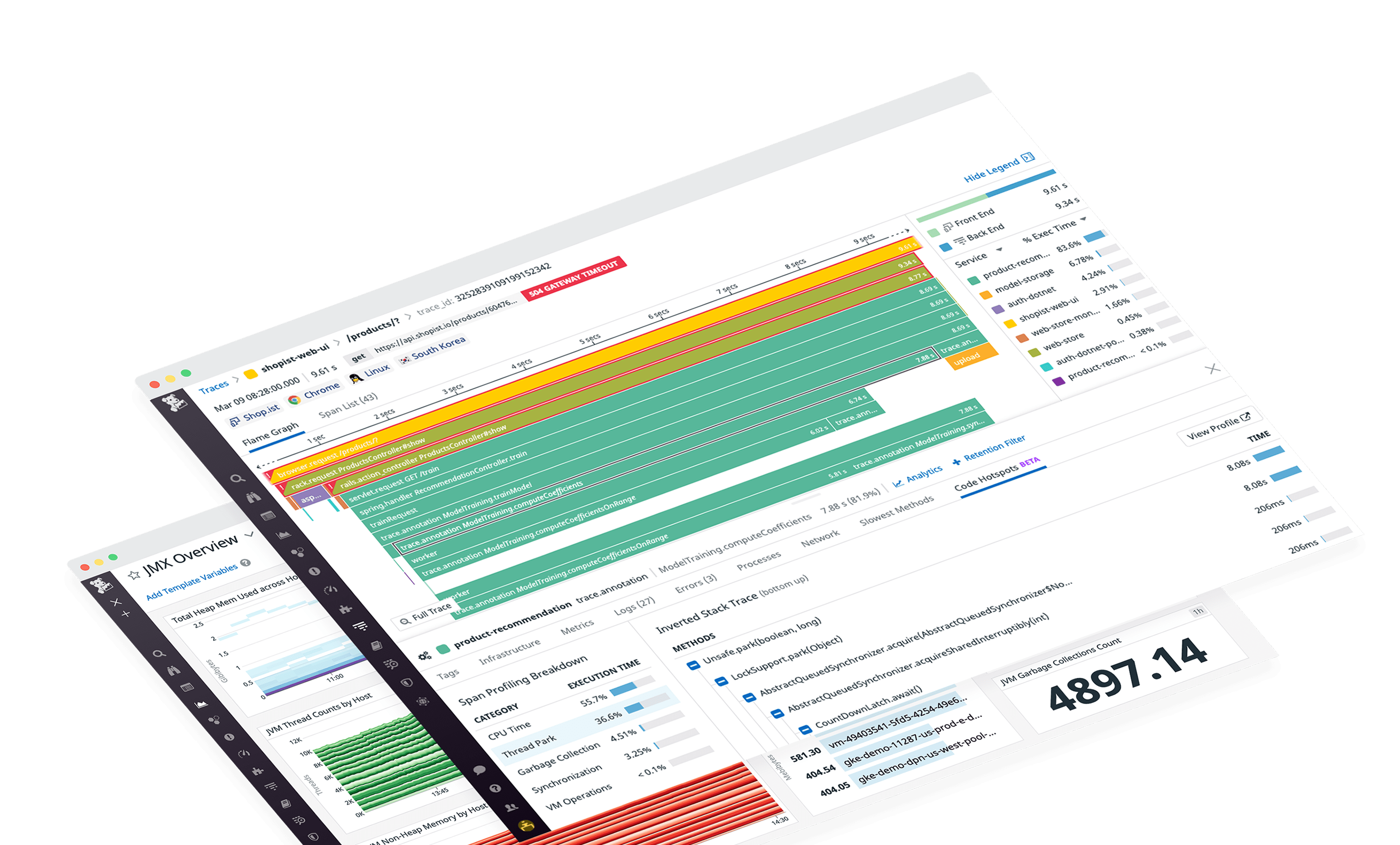The image displays a digital screen capture, likely from a laptop or computer, showing a spreadsheet or information display with overlays of two main sections, one overlapping the other and both slightly off-center. At the top of the screen capture, a blue border outlines the section labeled "traces" and "shop list web." Below this, there are yellow and light green bar graphs, though the text within these colored sections is difficult to read. The top horizontal axis shows time in seconds. Notable labels such as "browser request products," "rack request," "worker," and "trace annotation" are seen within these sections.

On the left side of the screen, a black border features icons typically found on a website interface, adding to the complexity of the visual. In the upper left gray border, small red, yellow, and green dots are visible. A prominent red box within the display contains the text "504 Gateway Timeout."

At the very bottom of the screen, against a black background, a numeric value "4,897.14" is clearly readable, labeled as "JVM garbage collections count." This combination of details suggests that the user is monitoring web activity, possibly through a browser like Google Chrome, with additional tabs open including "Linux," "Shop IST," and "South Korea," hinting at varied browsing activity or tasks.